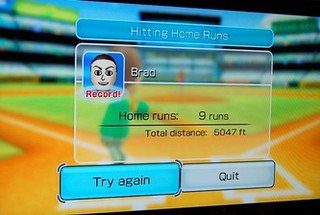In this rectangular image, we see a screen displaying a video game, partially framed by black edges from the surrounding room visible in the upper right and lower right corners. The screen predominantly features an orange backdrop with a green interior representing a baseball field. The perspective is from the batter's viewpoint, with the field enclosed by stands filled with cheering fans. At the top of the screen, text indicates the context of "hitting home runs."

In the upper left corner, an image of a player's face is shown, with the name "Brad" displayed alongside. Brad's character has brown hair and brown eyes. Below his image, it reads "Record!" indicating a significant achievement. Brad has scored 9 home runs, with a total distance of 5,047 feet.